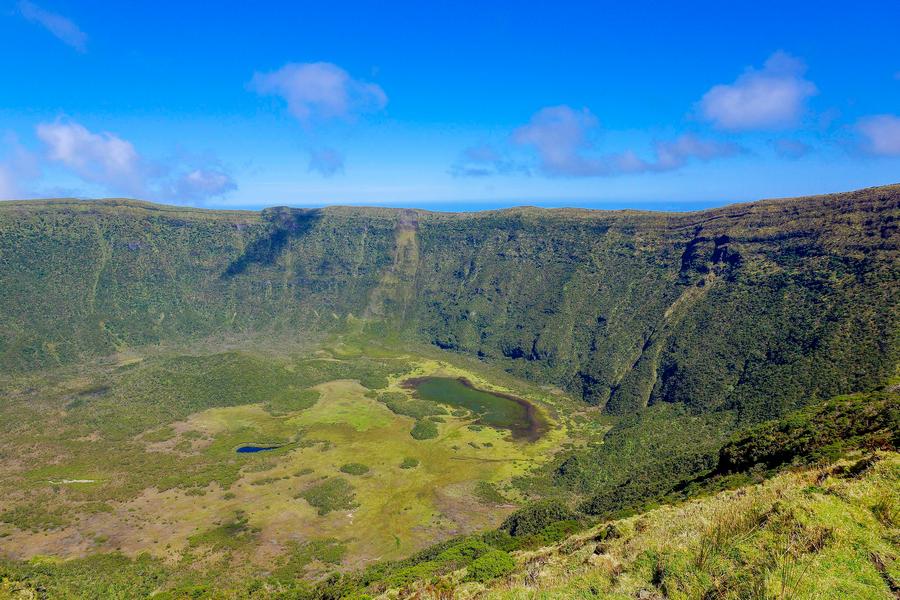The image captures a vibrant and picturesque caldera, a type of valley formed by a collapsed volcanic mountain. The scene is dominated by the lush green vegetation that carpets both the higher rocky edges and the lower central area, interspersed with patches of yellow-brown grass. A striking feature in the center is a small blue pond surrounded by greenery, adding contrast to the landscape. The horizon is marked by the high, uneven edges of the caldera, and you can detect low-growing shrubs scattered along these slopes. The backdrop is a stunningly clear blue sky, transitioning to white near the horizon, adorned with a few small, wispy white clouds dispersed evenly across the view. The overall impression is of a serene and richly colored natural haven, likely captured in the springtime.